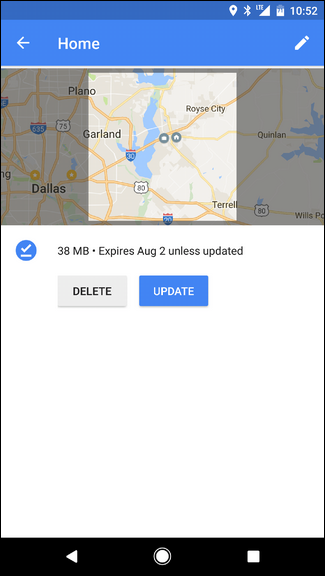The image is a color screenshot, taken at 10:52, of a smartphone in profile format. The phone shows around 80% battery life left and full reception. The Bluetooth and map features are activated, as indicated by the icons in the top right corner. The screenshot displays the smartphone's home screen with a visible back option, revealing a Google Maps interface. The map features a focused section, highlighted in a brighter square, depicting a specific area northeast of Dallas, including Garland and Royce City. The rest of the map appears dimmer. Beneath this map section, there is a note stating "38 megabytes expires August 2 unless updated." Two app options are available below: a beige "DELETE" button with black uppercase lettering, and a blue "UPDATE" button with white uppercase lettering.